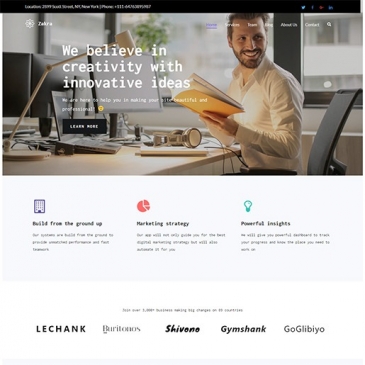The image has a dark black border at the top, featuring some white text. Below this border, there is a picture of a man seated at a desk. He has a mustache and a thin goatee with a beard. The man is wearing a long-sleeved white dress shirt without a tie, and he is sitting in a black chair with the backrest bent at a curved angle. Behind him, there are windows through which a tree is visible.

In white text overlaid on the window area, the message "We believe in creativity with innovative ideas" is displayed. The man is holding a manila folder in his hand. On the desk in front of him, there is a set of headphones, a computer monitor, and a lamp with a long bar connecting to its base. There is also a black rectangular button that reads "Learn More."

The image further includes three paragraphs of text situated on the left, middle, and right sides of the image, although this text is too blurry to read. At the bottom of the image, several brand names are listed: LeChink, Chavin, Jim Shank, and Go Glibio.